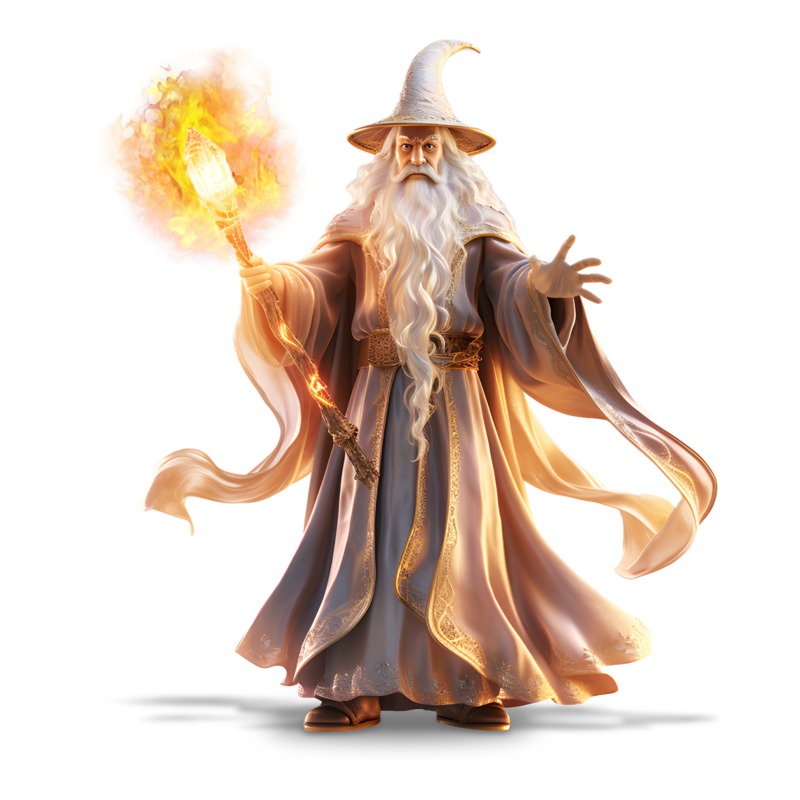This image depicts a detailed illustration of a wizard, reminiscent of fantasy characters from Harry Potter or Dungeons and Dragons. The wizard is an older white man with a long, flowing white beard and matching mustache that extend past his belt. His elaborate attire includes a large, curved, pointy hat with a circular brim, and a magnificent robe that appears white with gold trim and intricate designs along the seams. The robe has long, flowing sleeves, adding to the grandiose appearance. He wears brown boots visible beneath the hem of his robe. In his left hand, he holds a wooden staff adorned with a glowing gem or crystal, which emits a vivid, fiery red energy, casting a warm yellow and orange light onto his robes. There is a plastic-like, beautifully crafted depiction of fire emanating from the staff, which suggests magical power. The background of the image is plain white, emphasizing the wizard figure without any distractions.